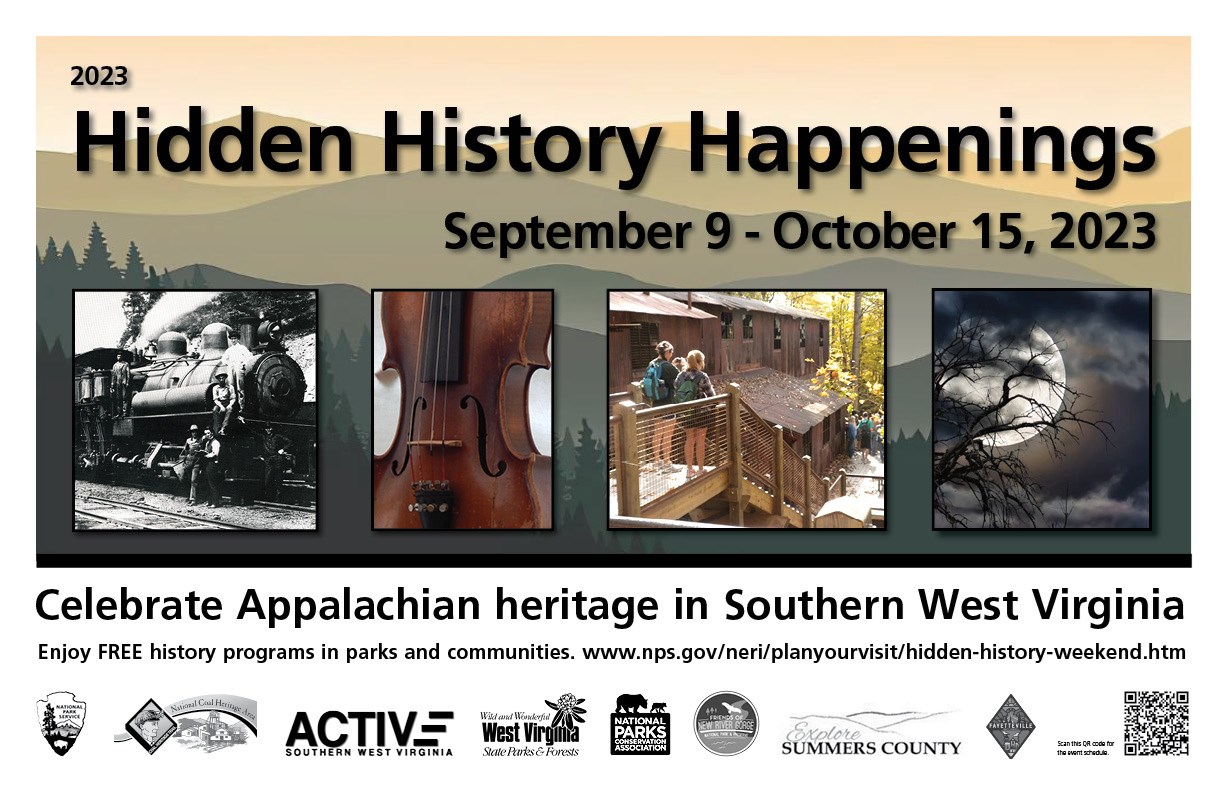The flyer is promoting an event titled "2023 Hidden History Happenings" and runs from September 9th through October 23rd. The background features a stylized hilly landscape with forest trees at the bottom, transitioning from greenish-gray to cream, with the sky a very light beige. Black text at the top left reads "2023," and the event title "Hidden History Happenings" stretches across the top. Below, right-aligned text notes the event dates, "September 9th - October 23rd, 2023."

The flyer includes four square images: the first is a black and white train, the second is a close-up of a violin, the third shows two girls on steps taking a picture in an empty barn, and the fourth photo captures the night sky with the moon peeking behind a dark, dry tree.

Underneath the images, a white rectangle states, "Celebrate Appalachian heritage in Southern West Virginia." The bottom section of the flyer contains multiple sponsor logos and features a QR code in the lower right corner.